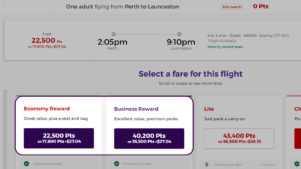In this image, you see text detailing flight reward options. There is one adult flying from the North to Lanchestone. The options include an economy reward at 2,500 points and a business reward at 40,200 points. The displayed fare information is primarily in shades of purple, orange, white, and black. The image contains no additional details beyond these text elements and color schemes.